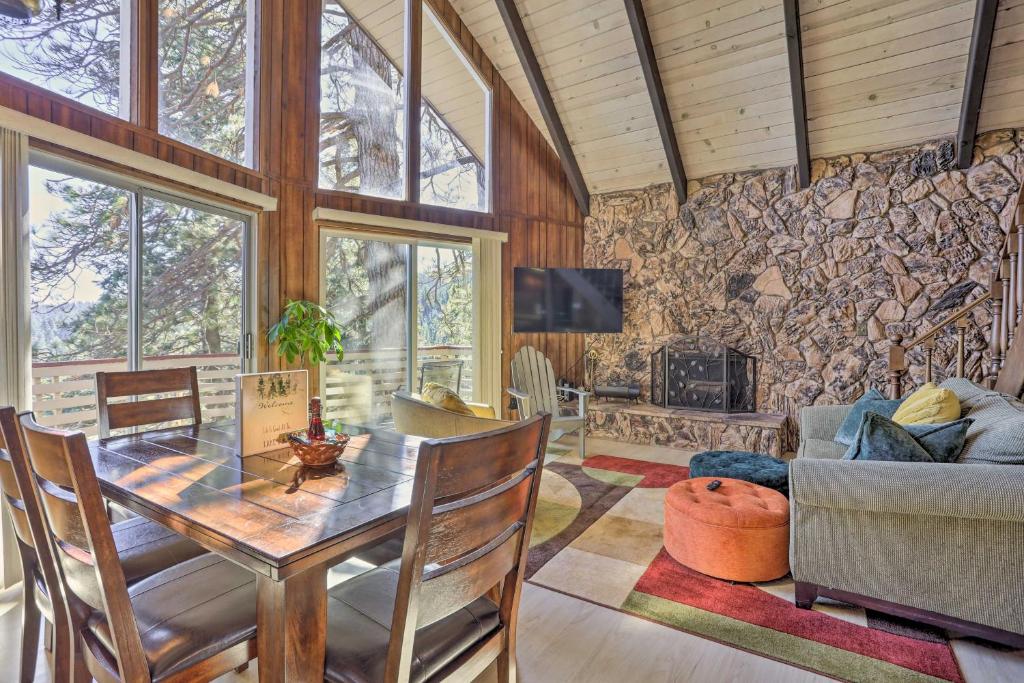This image captures the interior of a charming, farmhouse-style cabin with a blend of rustic and modern aesthetics, taken from a diagonal angle to showcase multiple areas. To the left, a traditional dark wooden dining table with a centerpiece of a card and bowl holding a sauce bottle is surrounded by four wooden chairs. Behind the table, large paneled windows framed by dark wooden paneling reveal a view of towering trees and a porch. The right side of the room features a wide stone wall with a fireplace, above which hangs a widescreen television. To complement the farmhouse look, a gray Adirondack chair sits under the TV. The area also exhibits a geometric, abstract rug with two circular ottomans, placed next to a cozy gray couch adorned with large pillows. High, vaulted ceilings with white pine wooden planks and beams add to the spaciousness. On the right side of the image, a staircase leads to an upper level. This well-lit cabin in the woods merges the warmth of rustic elements with modern comforts, creating an inviting and picturesque living space.